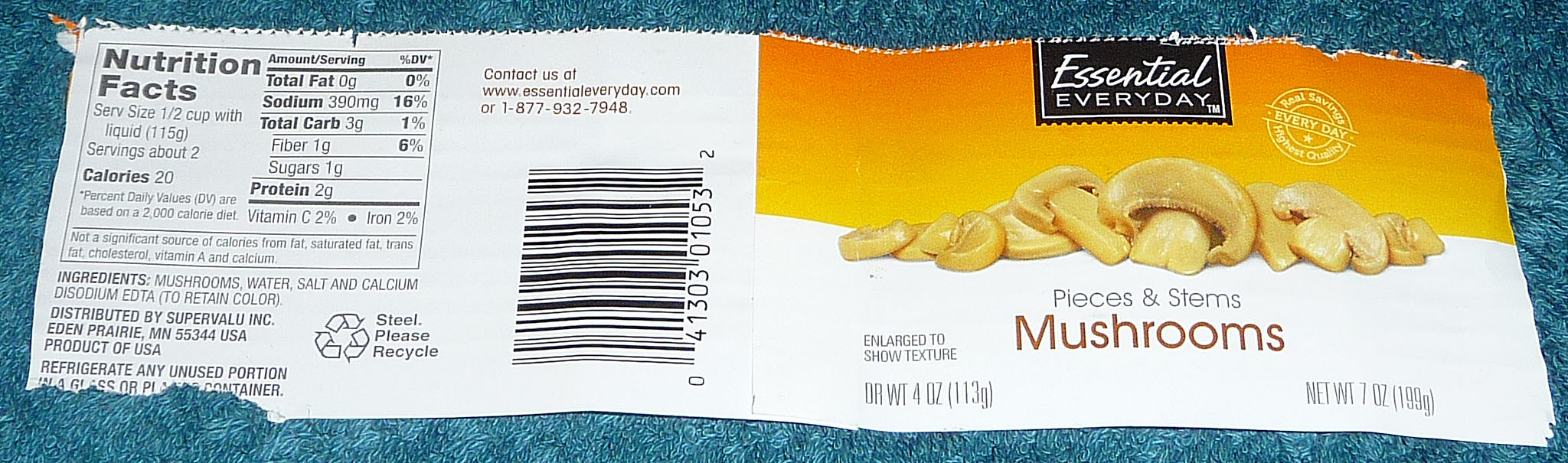The image showcases the label of an Essential Every Day brand mushroom package, meticulously laid out on a light blue, textured countertop. The top half of the label is showcased in an eye-catching orange with a centered black square that prominently displays "Essential Every Day" in white text. The bottom half transitions to a clean white background, featuring a detailed photograph of sliced mushrooms, clarified with the text "pieces and stems mushrooms."

The reverse side of the label is also visible and includes comprehensive nutritional information such as:
- **Total Fat**: 0g
- **Calories**: 20
- **Serving Size**: 1/2 cup
- **Sodium**: 390mg
- **Total Carbohydrates**: 3g
- **Dietary Fiber**: 1g
- **Sugars**: 1g
- **Protein**: 2g

It also lists the ingredients: Mushrooms, Water, Salt, and Calcium Disodium EDTA to retain color, indicating that these mushrooms are preserved in water. The barcode is present alongside the nutritional facts, rounding out the thoroughly detailed presentation of the package label.